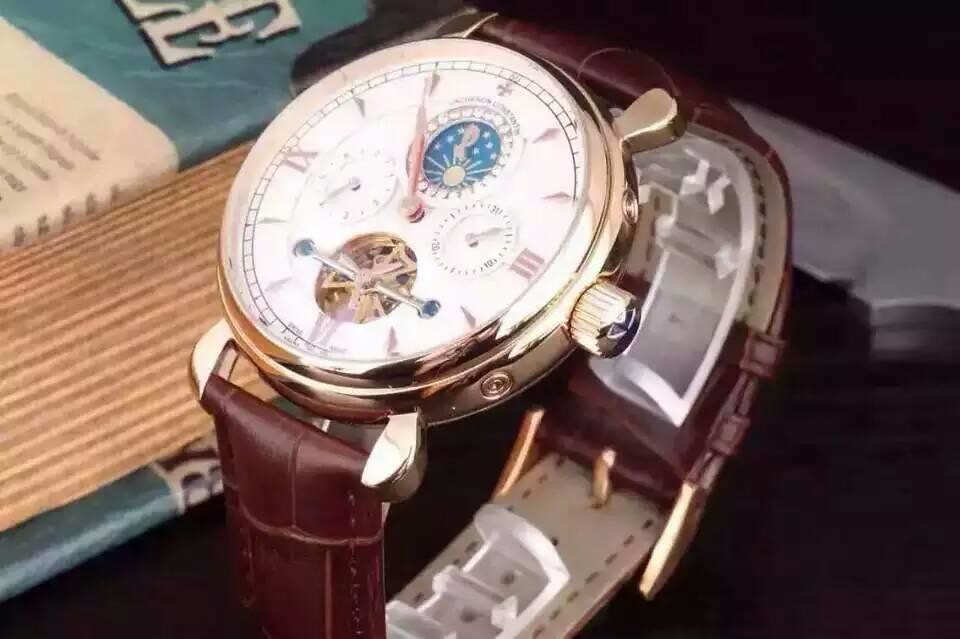The image is a meticulously crafted advertisement for an exquisite wristwatch, prominently centered in a horizontal layout. The focal point of the composition is the watch itself, which rests elegantly atop several books positioned behind it and slightly to the upper left. The watch boasts a rich brown leather band with a comfortable white inner lining, exuding a classic yet refined aesthetic. Its bezel and stem are adorned in a lustrous gold color, harmoniously complementing the watch’s face, which is a pristine white.

The watch face is detailed with Roman numerals, also in gold, enhancing its timeless appeal. At the 12 o'clock position, an open circular segment reveals a starry sky and a bright sun, indicative of the day-night cycle functionality. Similarly, another open section at the 6 o'clock position provides a glimpse into the intricate internal mechanisms of the watch, showcasing the craftsmanship that lies within. Flanking these features, two additional circular dials are situated at the 3 o'clock and 9 o'clock positions, each housing sleek needle indicators. The dials likely serve as a timer and another yet undetermined function, adding to the watch’s versatility and utility.

The hour and minute hands share the same opulent gold hue, ensuring clarity and elegance in time-telling. This carefully detailed wristwatch, set against the backdrop of scholarly books, conveys a sense of sophistication and intellectual charm, making it a perfect blend of style and functionality.